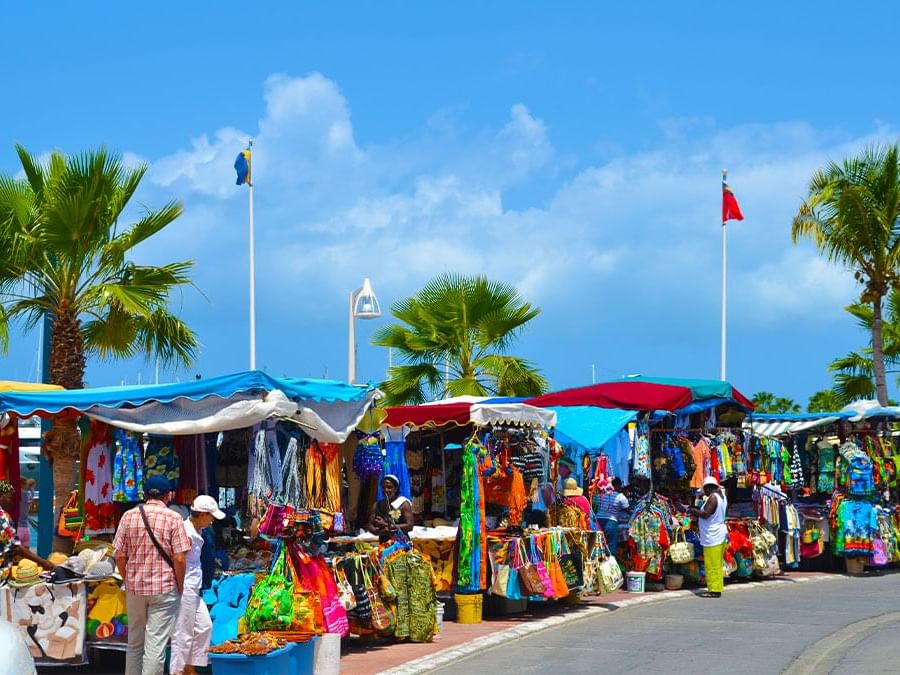This landscape-format photograph captures a vibrant outdoor market in a tropical, seaside location, likely somewhere in the Caribbean, as suggested by the palm trees in the background. The scene is bathed in bright sunlight with a few distant clouds dotting the clear sky. The market is bustling with stalls draped in colorful fabric canopies, providing shade for the array of vividly colored goods on display. These include tie-dye and Hawaiian-style buttoned shirts, handbags, hats, shorts, and other fabric-based items, all in striking hues of red, orange, green, and blue.

The market stalls are arranged along a curved road, creating a lively and bustling atmosphere. People of color, both customers and vendors, animate the scene, engaging in lively exchanges and browsing the vibrant merchandise. Two specific tourists, donning baseball caps, are seen examining items at the forefront of the first stall.

In the background, the photograph hints at a seaside setting, with the mast tops of boats peeking above the horizon. Two flagpoles stand proud, one flying a blue flag and the other a red flag, adding to the colorful tableau. A single street light and a lantern protrude above the stalls, blending into the tropical ambiance of this bustling market bazaar.